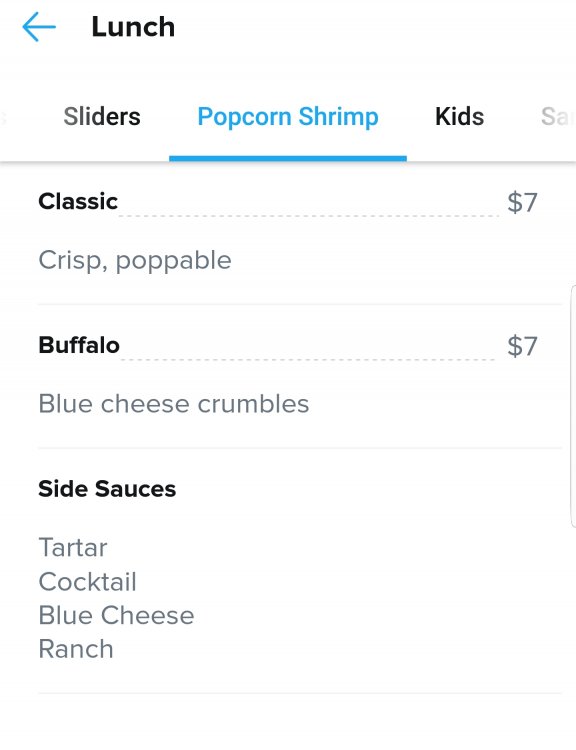This image appears to be a screenshot from a mobile app, featuring a menu with a white background. At the top left corner, there is a blue left-pointing arrow. Adjacent to this, the word "Lunch" is displayed in black text. Directly beneath this header, there is a navigation bar with three labeled sections: "Sliders" on the left, "Popcorn Shrimp" in the center (highlighted in blue), and "Kids" on the right (in black text). A blue underline emphasizes the "Popcorn Shrimp" section.

The detailed portion of the menu begins below this navigation bar. On the left side, under the "Popcorn Shrimp" category, there are a series of menu items listed vertically and in black text:
- Classic
- So Crisp
- Poppable
- Buffalo
- Blue Cheese Crumbles
- Side Sauces

Under "Side Sauces," there are additional items listed:
- Tartar
- Cocktail
- Blue Cheese
- Ranch

Corresponding to each main item listed on the left, prices are displayed on the right side of the screen in gray text:
- Classic: $7.00
- Buffalo: $7.00

There is a series of gray dots connecting the main menu items to their respective prices. The entire screenshot maintains a minimalist, clean design with light gray text for marginal elements like the sauce types. The overall presentation suggests that the app could be related to food ordering or nutrition tracking, such as something similar to MyFitnessPal.